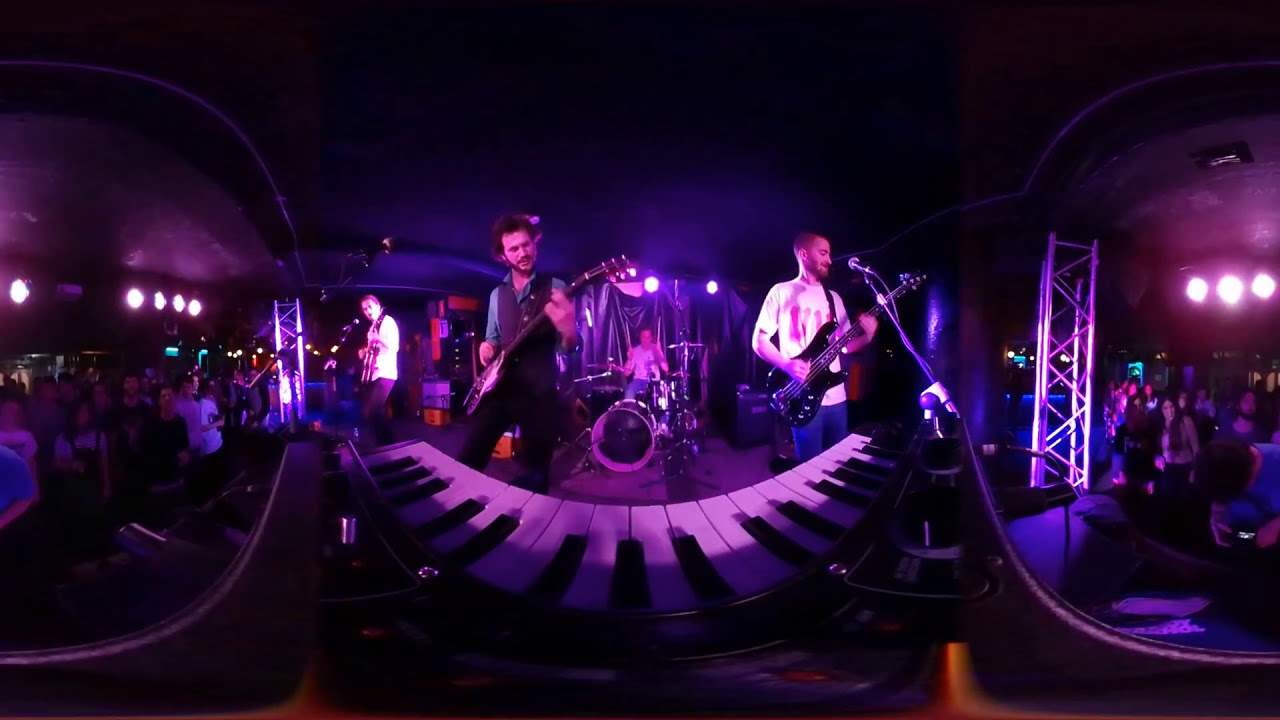This image captures a high-energy rock band performance in a dimly lit nightclub, accentuated by a purple hue that envelops the setting. The center stage is occupied by four casually dressed band members, clad in t-shirts, jeans, and casual attire reminiscent of an effortless yet stylish vibe. The ensemble includes two guitarists, a bassist, and a drummer with a transparent black drum set, complemented by a keyboard positioned at the front of the image.

The surroundings are equally engaging, with a fisheye lens adding a unique curvature to the edges of the rectangular frame, hinting at a dynamic and immersive atmosphere. The crowd flanks the stage on both sides, seemingly absorbed in the performance, though their positioning might suggest a video recording session. Overhead, round lights arranged in a horizontal row provide a stark white and purple illumination, while silver beams and a steel ladder rise from the floor to the ceiling, framing the energetic scene.

Each band member is vividly detailed: one guitarist in a white shirt with a black guitar strap, another sporting a gray vest over a blue shirt, and the drummer in a white shirt and blue jeans. Together, their casual yet upper-class look echoes bands like The Strokes, promising a blend of refinement and rock 'n roll authenticity.